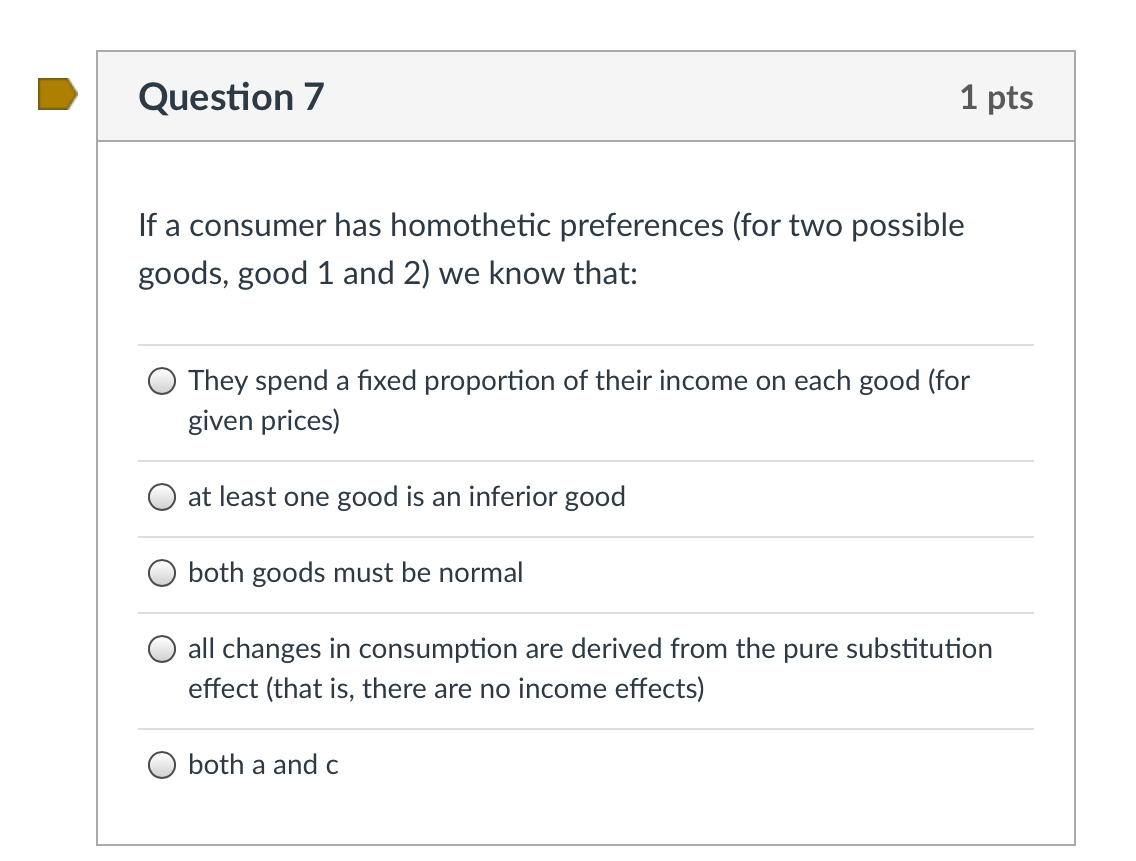The image features a themed multiple-choice question titled "Question 7, One Point." It presents a query about a consumer's homothetic preferences for two possible goods, labeled Good 1 and Good 2. The question is followed by five distinct answer options:

1. They spend a fixed proportion of their income on each good for given prices.
2. At least one good is an inferior good.
3. Both goods must be normal.
4. All changes in consumption are derived from the pure substitution effect; that is, there are no income effects.
5. Both A and C.

The question is enclosed in a square box with a black border, ensuring it stands out prominently. The background within the box is predominantly white with black text for high contrast and readability. At the top left corner of the box, there is a golden, tag-shaped indicator designed to help users easily keep track of their progress. The layout and dot navigation features suggest that this question could be part of an interactive quiz or examination, likely completed on a computer, where selections can be made using a mouse.